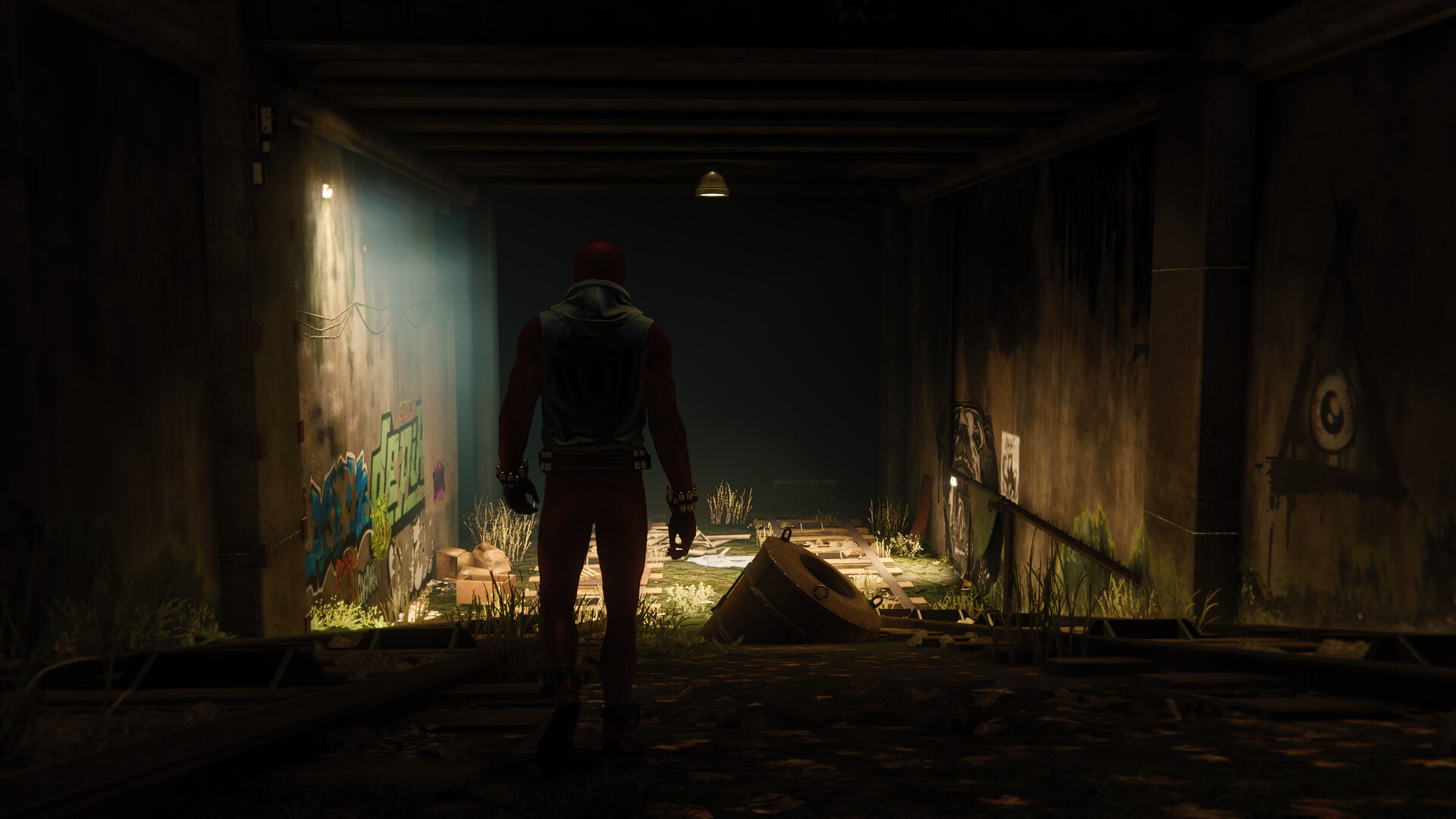This screenshot depicts a scene from a video game set in a dimly lit urban environment. The lighting emanates from a source atop the left side of a concrete wall, casting a beam that illuminates a sloped walkway in the background. In the foreground, a character stands slightly left of center with his back to the viewer. He is dressed in a distinctive red leotard outfit, complemented by a black leather vest and black leather gloves adorned with spikes. His head is covered by a red ski mask, reminiscent of Spider-Man's attire. He appears to be observing an area beneath a bridge-like structure. The surrounding environment features high concrete walls on both sides, each adorned with vibrant graffiti. The ceiling above consists of metal grates, adding to the gritty, industrial feel of the scene.